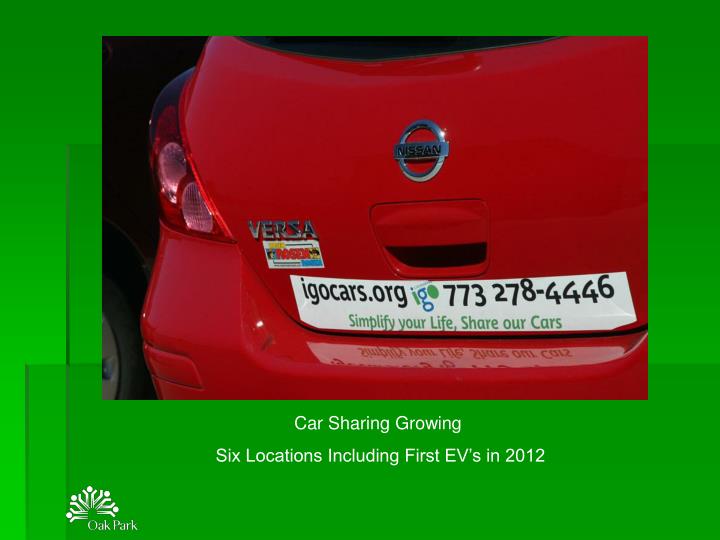This advertisement for car sharing features a bright red Nissan Versa positioned against a vibrant green background. The photograph shows the back of the car, highlighting the trunk handle, the Nissan logo, and the Versa badge. A bumper sticker prominently displays the website "igocars.com," followed by the phone number 773-278-4446, with the slogan "Simplify your life, share your cars" in green text beneath it. Towards the bottom of the image, a white stylized logo of four people in a circle, with accompanying text identifying 'Oak Park,' is visible. Running horizontally along the lower third of the advertisement, the text reads: "Car sharing growing: six locations including first EVs in 2012."